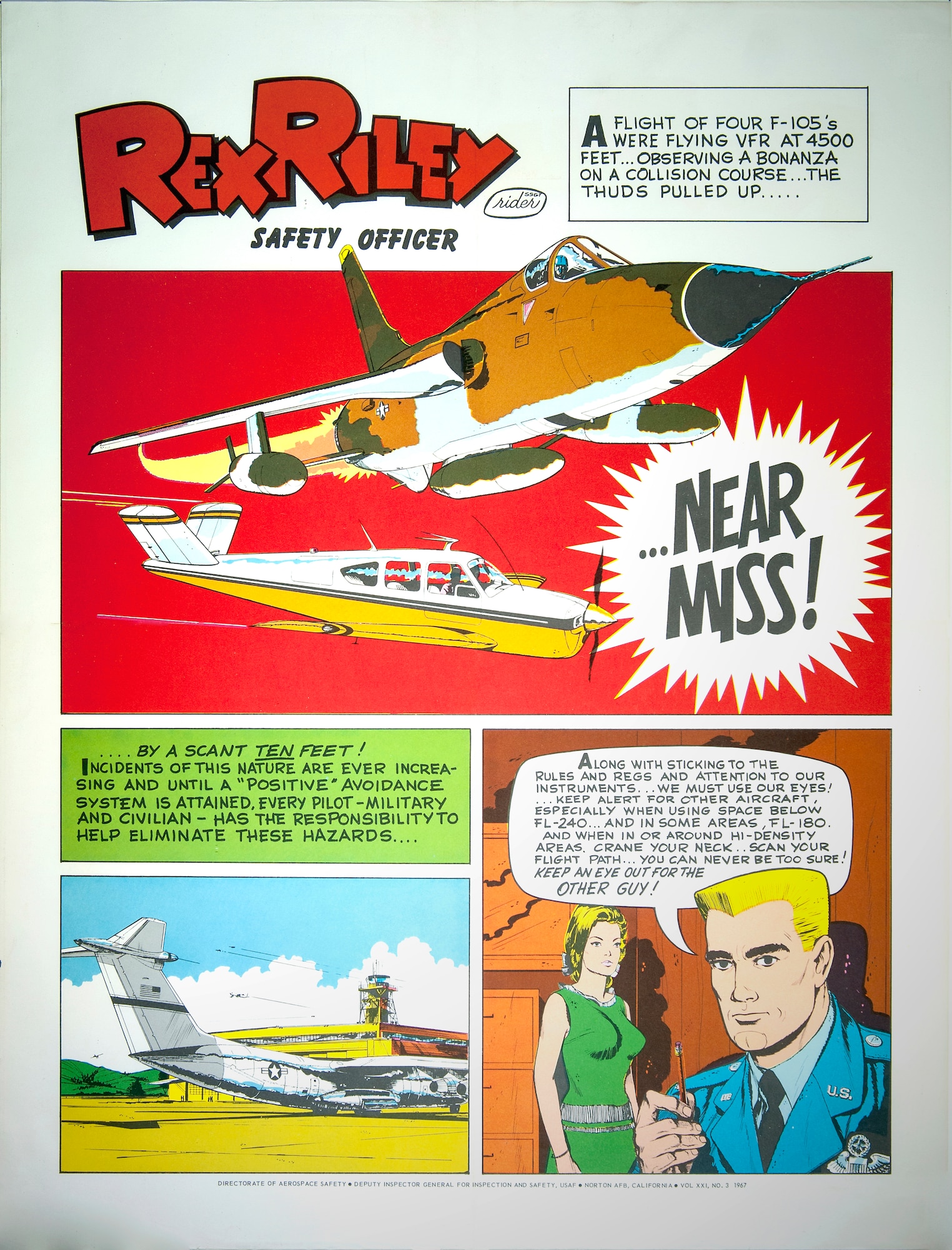This image is a detailed page from an old-fashioned comic book titled "Rex Riley, Safety Officer." The page features four colorful panels arranged in a classic comic book style. At the top of the page, there's prominently red-trimmed black text declaring "Rex Riley, Safety Officer."

The top right panel carries a narrative block that reads, "A flight of four F-105s were flying VFR at 4,500 feet observing a bonanza on a collision course. The thuds pulled up..." This panel features an illustration of an F-105 narrowly missing a smaller aircraft, possibly a Cessna, with the phrase "Near Miss" highlighted in a jagged white circle.

The second panel illustrates an airplane safely on the ground accompanied by the text, "...by a scant 10 feet. Incidents of this nature are ever increasing until a positive avoidance system is attained. Every pilot, military and civilian, has the responsibility to help eliminate these hazards."

In the bottom right panel, the comic shifts to a depiction of Rex Riley, a blonde crew-cut U.S. Air Force officer, engaged in conversation with a woman dressed in green. The woman, with her prominent features, appears to be listening attentively as Rex Riley emphasizes the importance of "watching out for the other guy," encapsulating the core safety message of the comic.